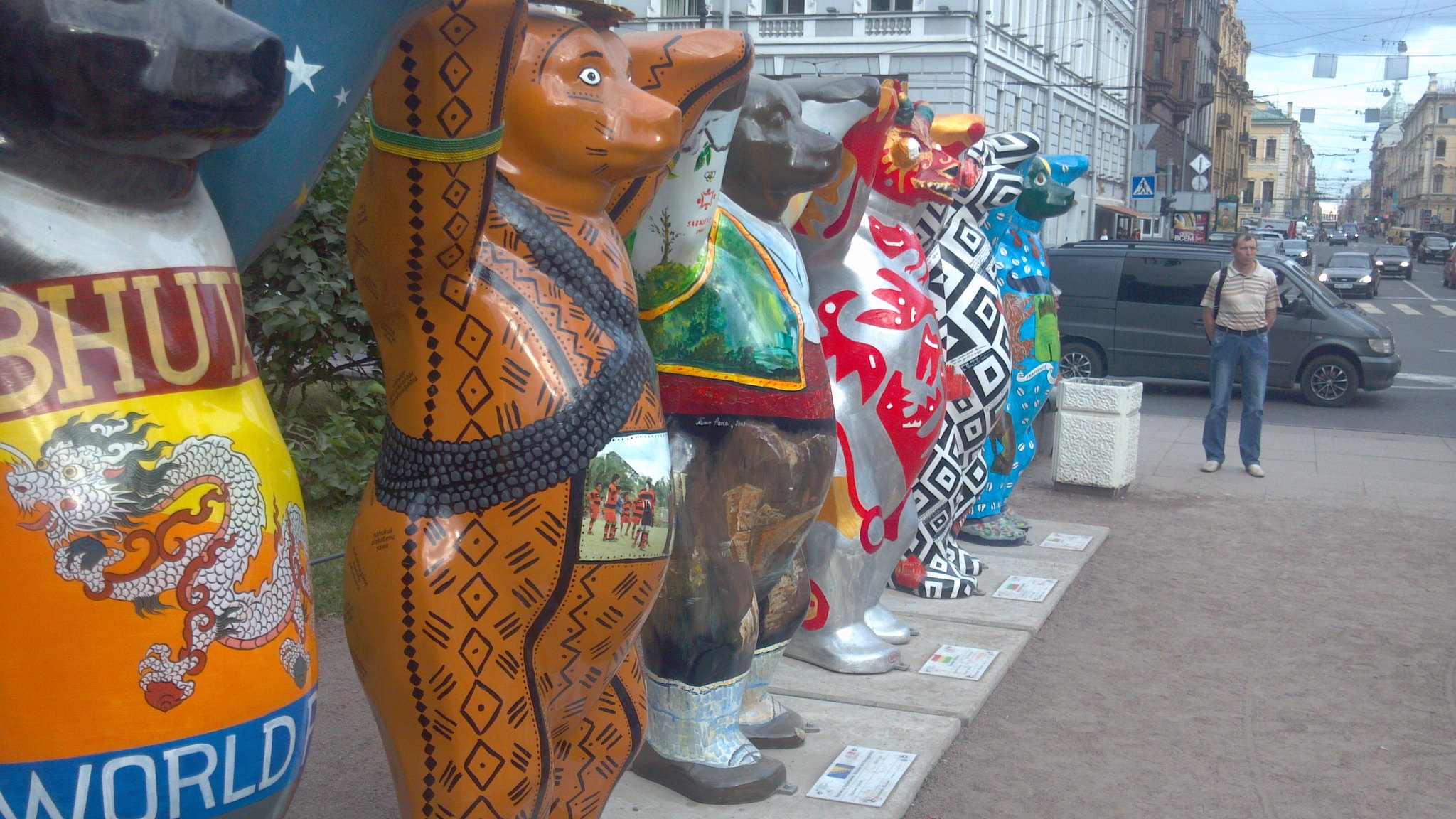This photo captures a vibrant city street, with various buildings stretching into the distance. In the foreground, a row of six large, intricately painted bear sculptures stand on a stone tablet placed on stone pavement. Each bear displays unique and vivid designs. The bear on the far left features a Chinese dragon on its stomach, set against a yellow background, with the words "B-H-U-T" inscribed on top and "WORLD" at the bottom, in white text on a blue background. Next to it, an orange bear showcases a black tribal design and white eyes. Another bear has a forest scene painted on its shirt. Following that, a silver-bodied bear with red decals and a red head stands prominently. The subsequent bear displays a geometric pattern of black and white shapes. All the bears are posed with their arms raised above their heads, seemingly holding hands. Each bear has a plaque at its base, potentially indicating the specific country or city they represent. In the background, a man dressed in blue jeans, a tan and brown striped shirt, and carrying a backpack stands near a green van. The scene exudes a sense of bustling urban life under clear weather conditions.